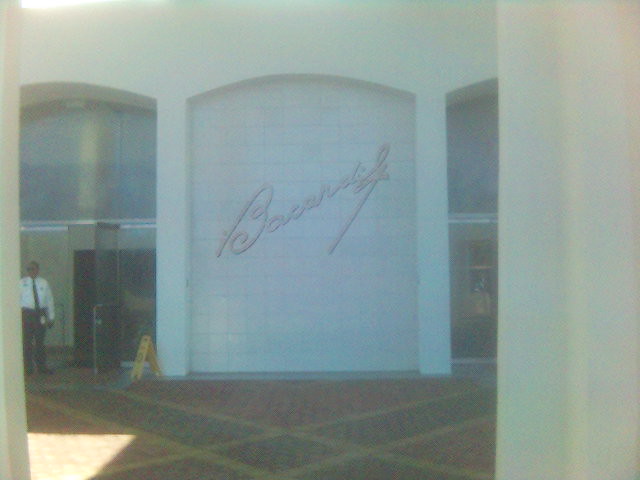This image, albeit overexposed and out-of-focus, presents a hazy view of the interior of a room. Dominating the center of the photograph is an upward-angled script written in a light pink hue, seemingly conveying a phrase related to "life," though the exact wording remains indiscernible due to the extremely low contrast. The foreground features a distinctive floor pattern comprising crisscrossed tiles in black with white trim, punctuated intermittently by touches of red.